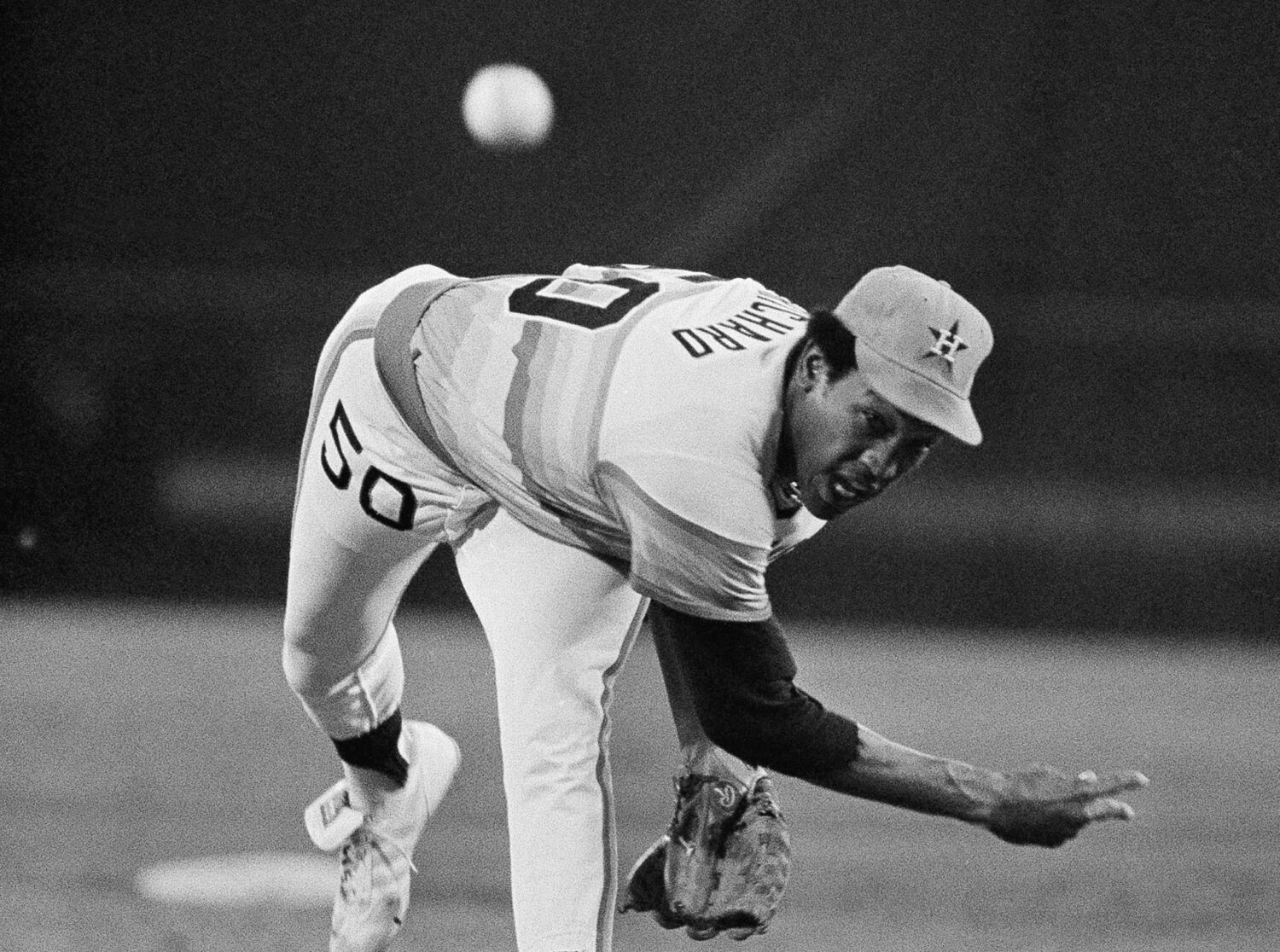This is a black and white, horizontally-oriented photograph depicting an African-American pitcher from the Houston Astros in mid-action during a game. The image, grainy and atmospheric, captures the precise moment immediately after he has thrown the baseball, which is seen in mid-flight towards the top center of the frame. The pitcher is bent over, his right leg raised, and his throwing arm arched all the way down to the lower right, emphasizing the momentum and force of his pitch. He is attired in the distinctive Houston Astros uniform: a white baseball cap with an "H" on it positioned over a dark-colored star, white pants, white sneakers, a dark long-sleeved shirt underneath a short-sleeved shirt featuring rainbow stripes and the number 50 prominently displayed on both his shirt and thigh. His glove is on his left hand, and his jersey partially reveals the name ending in "C-H-A-R-D" with a visible zero below. The background is blurred and dark, suggesting a night game, with indistinct structures resembling bleachers adding to the stadium ambiance.